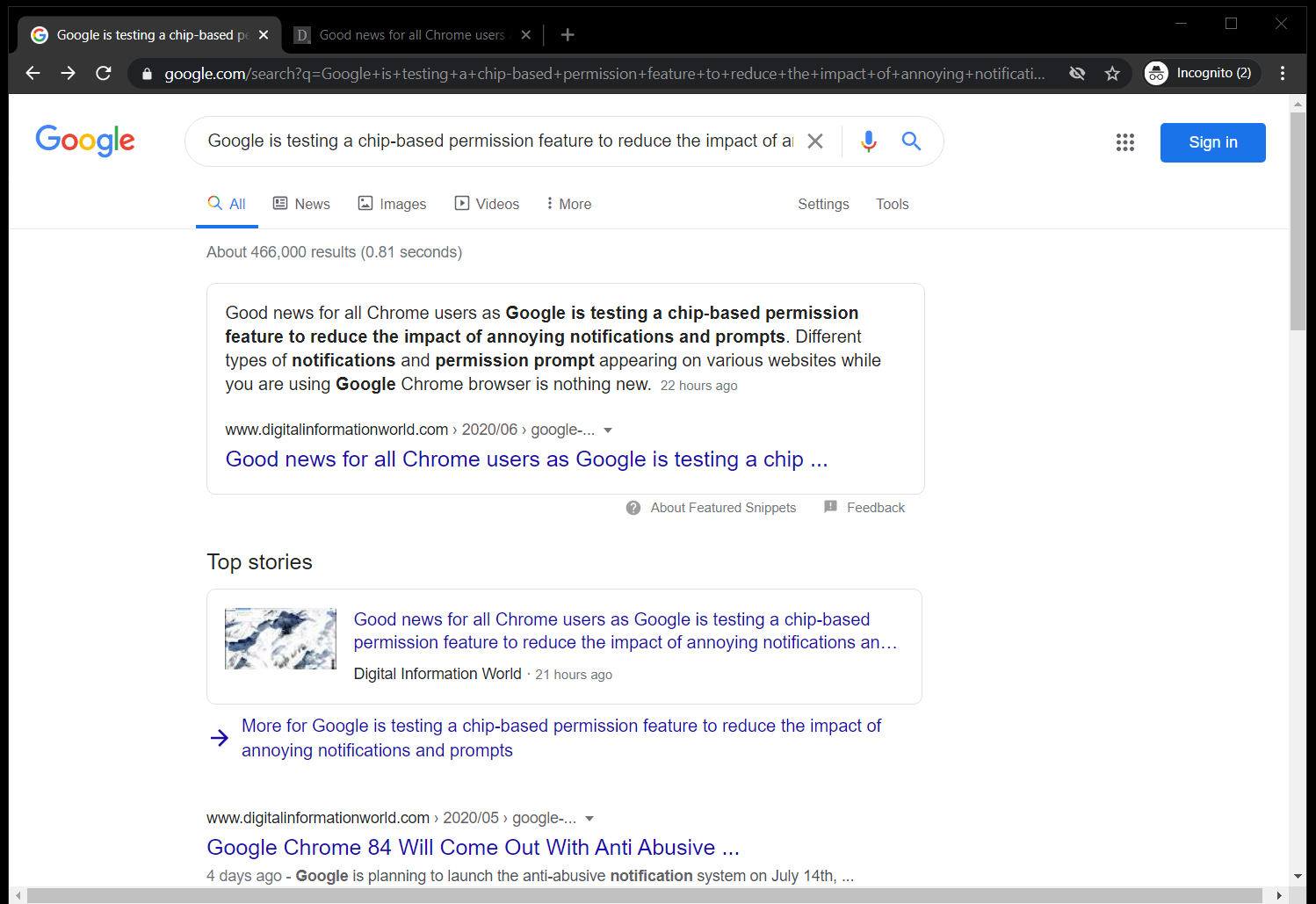The image shows an open incognito window in the Google Chrome browser. The search query entered is "Google is testing a chip-based permission failure to reduce the impact of a" which seems cut off. The top search result highlights a news article stating, "Good news for all Chrome users as Google is testing a chip-based permission feature to reduce the impact of annoying notifications and prompts." The summary mentions that various notifications and permission prompts appearing on websites in Google Chrome are being addressed by this new feature. The article was updated 22 hours ago and can be accessed by clicking the link.

Additionally, the search results indicate there are about 466,000 results generated in 0.81 seconds. The “Top Stories” section features the same article from Digital Information World, with an option to view more related stories. Another article from the same source below reads, "Google Chrome 84 will come out with anti-abusive...", suggesting further protective measures in upcoming Chrome updates. The user appears to be researching how Google Chrome plans to enhance user protection against intrusive notifications and pop-ups.